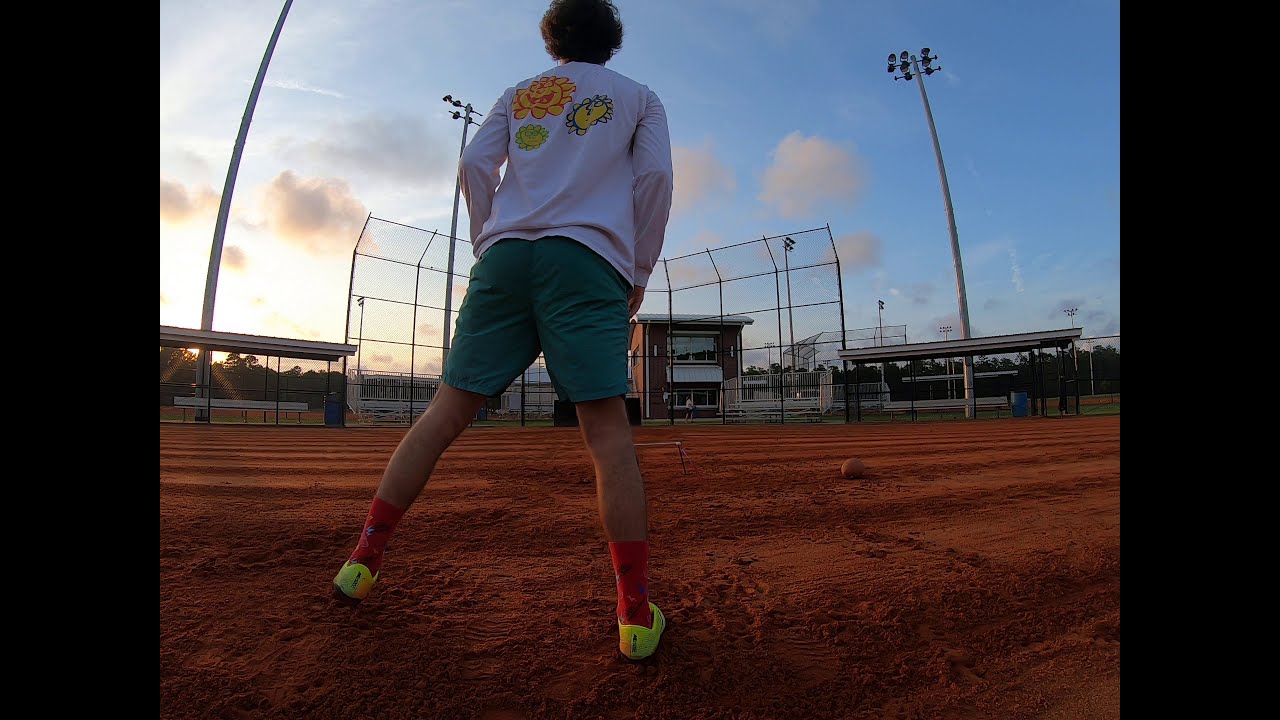The image captures a tranquil moment at dusk on a baseball field, framed by thick vertical borders. The sky is a light blue, punctuated by sporadic white and gray clouds, as the sun begins to set. The baseball field itself is a sandy brown dirt, with crisp white lines marking its layout. Central to the scene is a person dressed in a white long-sleeve shirt adorned with floral graphics on the back, green shorts, patterned red socks, and neon yellow cleats. They stand alone, facing away, with a brown ball slightly ahead of them. In the distance, a silver chain-link batter's cage stands empty, with a two-story brick building looming behind it. The field is sparsely populated, with a solitary figure barely discernible near the fence. Tall lamp posts, equipped with multiple spotlights, tower over the scene, ready to illuminate the field as night approaches.